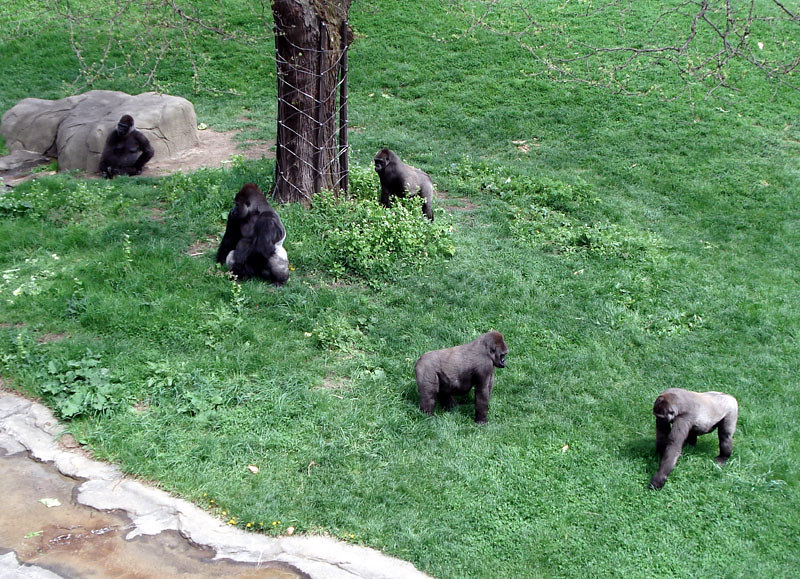This detailed daytime photograph depicts a gorilla enclosure, likely in a zoo, featuring five gorillas amidst a man-made environment. The setting includes a tree trunk wrapped with what appears to be silver wire or rope netting in a diamond pattern, designed for climbing. The grass in the enclosure is short and well-kept, unlike wild grass. To the left, an artificial rock outcropping and a boulder are visible, with one of the younger gorillas seated next to the boulder. The gorilla group comprises two younger silverback males, one of whom is sitting near the boulder while the other interacts with a female walking towards him through the deep green grass. The leading male, distinguishable by his presence and older appearance, is seated in front of the tree, while the second female walks toward the tree trunk. A portion of a brown dirt road is visible in the left forefront of the image, adding to the enclosure's landscaped appearance.